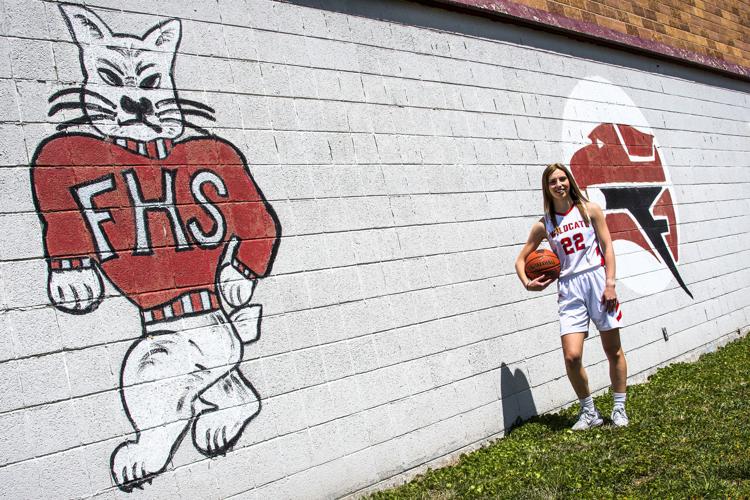The image is a rectangular landscape photograph featuring a young female basketball player, likely a teenager or in her early twenties, standing on green grass. She is wearing a sleeveless white jersey with red letters that spell "Wildcats" and the number "22," accompanied by matching shorts, white socks, and white tennis shoes. She has long, light brown or dark blonde hair, and she is smiling while holding a basketball in her right hand. Her left arm hangs straight by her side. 

Behind her is a gray cinderblock wall adorned with a cartoonish mascot of a white, upright-walking wildcat with three black whiskers on each side of its face. The wildcat mascot is dressed in a red sweater with the white letters "FHS" on it. Also visible on the wall is another circular symbol with red and black lettering. Above this cinderblock wall, in the upper right-hand corner of the image, a section of a brown brick wall is visible.